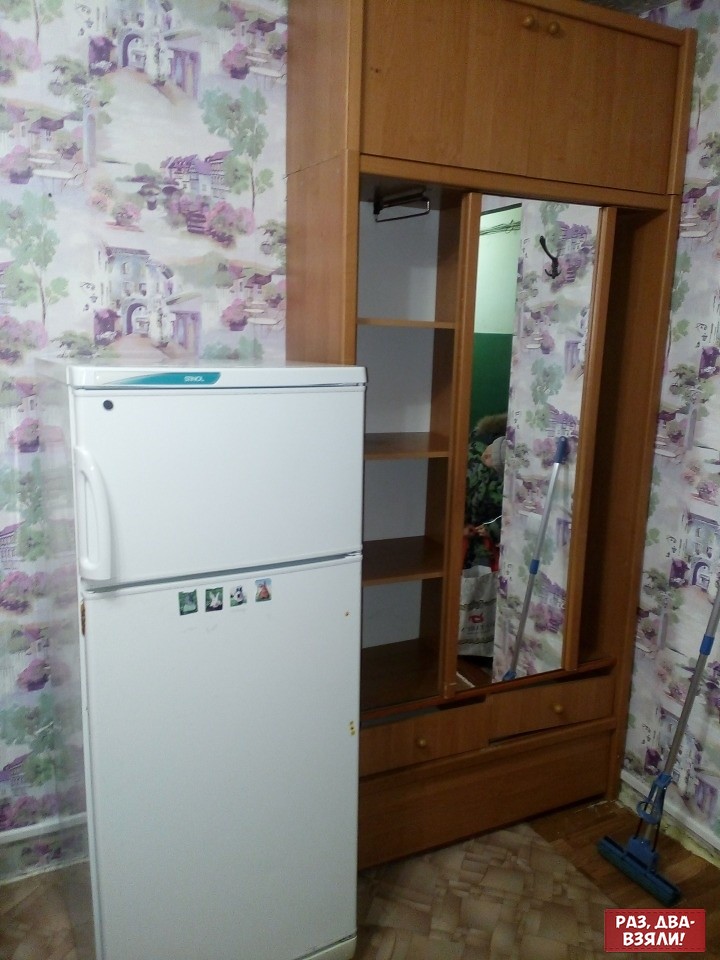This photo depicts the interior of a quaint and possibly vintage kitchen within someone's house. Central to the image is an old, apartment-sized white refrigerator adorned with four small magnets. The refrigerator features a freezer compartment with a horizontal door at the top, characteristic of older models.

To the right of the refrigerator stands a substantial wooden cabinet that combines the functions of a dresser and a closet. This piece includes drawers at the bottom, shelves, and a mirror in the middle, suitable for storing clothes and other items. The cabinet is described variously as having a pullout drawer on top and being designed to hang clothes.

Both walls, left and right, are covered with white wallpaper that features a pattern of purple flowers, buildings, and trees, creating a nostalgic ambiance. The floor below exhibits a dual-toned design: a section of brown-patterned carpet overlaying a wooden floor underneath.

A mop leans against the right wall, near the wooden cabinet. Reflecting in the cabinet's mirror is a glimpse of what might be another room and a coat hook, further adding to the cozy and lived-in feel of the space.